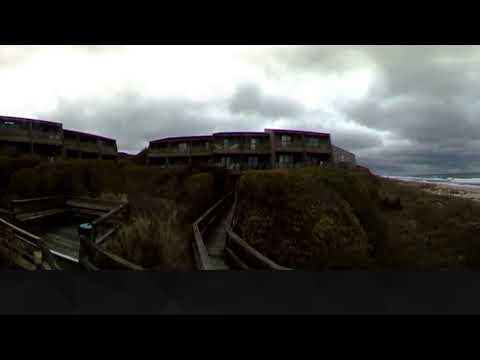The image captures a detailed, comprehensive view of a two-story gray-brown resort or hotel situated on a sloped hill covered in dark olive green and beige mossy grass. The landscape is portrayed in a color photograph taken from a drone, providing a panoramic perspective with the scene split into two combined photos—one viewing the building from the side and the other straight on. The building, segmented into five visible frames, features a wooden walkway and deck leading up to it, with an observation platform on the left made out of the same wooden structure. Wooden steps ascend towards the building, surrounded by greenery including bushes and some trees. The sky is filled with gray rain clouds, casting a gloomy atmosphere accentuated by some bright white light filtering through. The terrain to the right of the structure descends toward a narrow strip of ocean, where white waves lap at the shoreline. The beach and ocean glimpses, along with the surrounding grassy hill and vegetation, contribute to a serene yet somber coastal landscape.